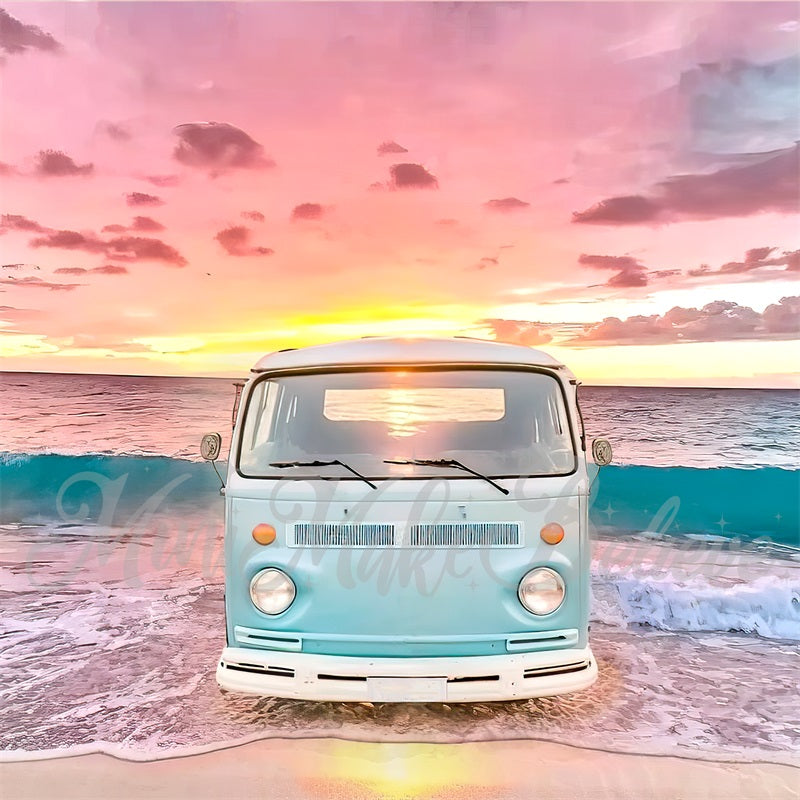The image depicts a charming vintage 1960s Volkswagen van positioned right at the edge of a beach where the surf meets the sand. The van has a distinct baby-blue or light blue, pearlized finish with a white roof, white bumpers, round white headlights, and pale orange blinker lights situated above. Two horizontal windshield wipers adorn its flat front. The vehicle also features two extended side mirrors and slatted radiator panels. It sits partially in the water with gentle waves foaming beneath its bumper and a larger turquoise wave curling behind it across the width of the picture.

The sky above is a mesmerizing blend of pale yellows, pinks, darker pinks, and hints of purples and blues, indicative of a vibrant sunrise or sunset. A streak of sunlight highlights the roof of the van, reflecting its soft glow onto the pink-tinted sand. The ocean mirrors the sky’s colors, displaying shades of turquoise, pink, and blue. The entire scene is suffused with a photorealistic quality enhanced by filter effects, giving the image an almost surreal, painterly appearance. In the lower third of the image, across the front of the van, there is a barely legible phrase in muted colors that reads, "many make believe."